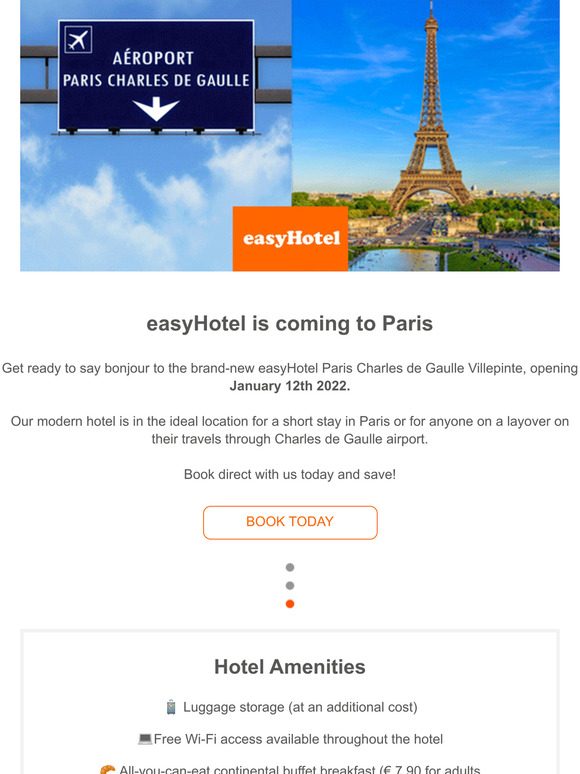This is a detailed caption for an image from the Easy Hotel webpage:

---

Screenshot of the Easy Hotel webpage's announcement for their new Paris location. The top section of the webpage features two photographs: one showing a sign for Paris Charles de Gaulle Airport, and the other depicting a distant view of the Eiffel Tower. Positioned between these images is the Easy Hotel logo, which has a striking orange background with white text, prominently capitalizing the "H" in "Hotel". 

The announcement text reads: "Easy Hotel is coming to Paris. Get ready to say bonjour to the brand-new Easy Hotel Paris Charles de Gaulle Villa Ponte, opening on January 12, 2022. Our modern hotel is in an ideal location for a short stay in Paris or for travelers on a layover at Charles de Gaulle Airport. Book directly with us today and save." 

Below the announcement, there is a pill-shaped bar with a white background and the text "Book today" in bold orange font. Further down, three colored dots serve as navigational indicators, followed by a section detailing the hotel amenities, which include: luggage storage available at an additional cost, free Wi-Fi access throughout the hotel, and an all-you-can-eat continental buffet breakfast priced at 7.90 euros for adults.

---